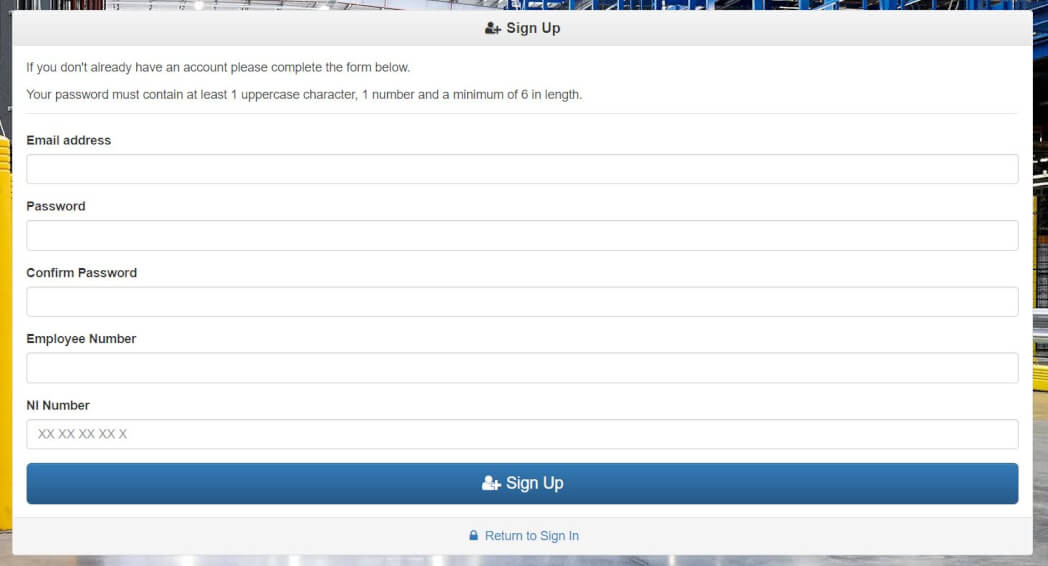The image depicts a website sign-up page with a clear and organized layout. At the top of the page, the header reads "Sign Up." Below the header, there is a message encouraging users who do not already have an account to complete the form provided. The form includes the following blank fields:

- Email Address
- Password, with a note that the password must contain at least one uppercase character, one number, and be a minimum of six characters in length
- Confirm Password
- Employee Number
- NI Number, which is pre-populated with the format "XX XX XX XX X"

Beneath these fields, there is a long blue rectangular button centrally positioned, labeled "Sign Up" with an icon of a person's silhouette and a white plus sign to its left. Directly below this button is a blue padlock icon accompanied by the text "Return to Sign In."

The image is clearly focused on the digital form and does not include any people, animals, plants, buildings, motorized vehicles, or bicycles. The simple and functional design highlights the essential elements necessary for account creation.